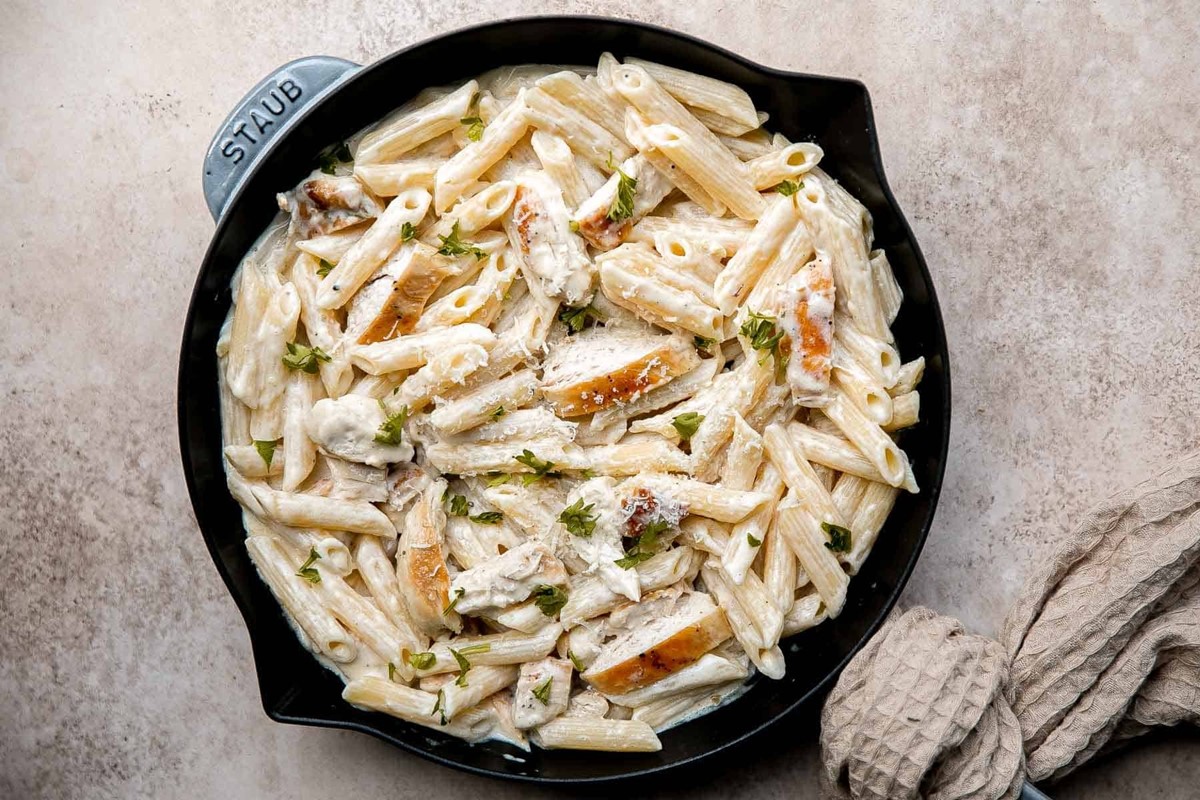The image shows an aerial view of a plate of penne pasta inside a black cast iron pot from the brand STAUB, identified by the engraved handle. The pot rests on a muted tan cream countertop. The pasta, smothered in a creamy white sauce, includes slices of chicken, garnished with green herbs, possibly parsley, and sprinkled with parmesan cheese. Additionally, slices of bread are interspersed with the pasta. The pot has a towel wrapped around its handle, suggesting it is hot. The dish appears untouched and ready to be served.